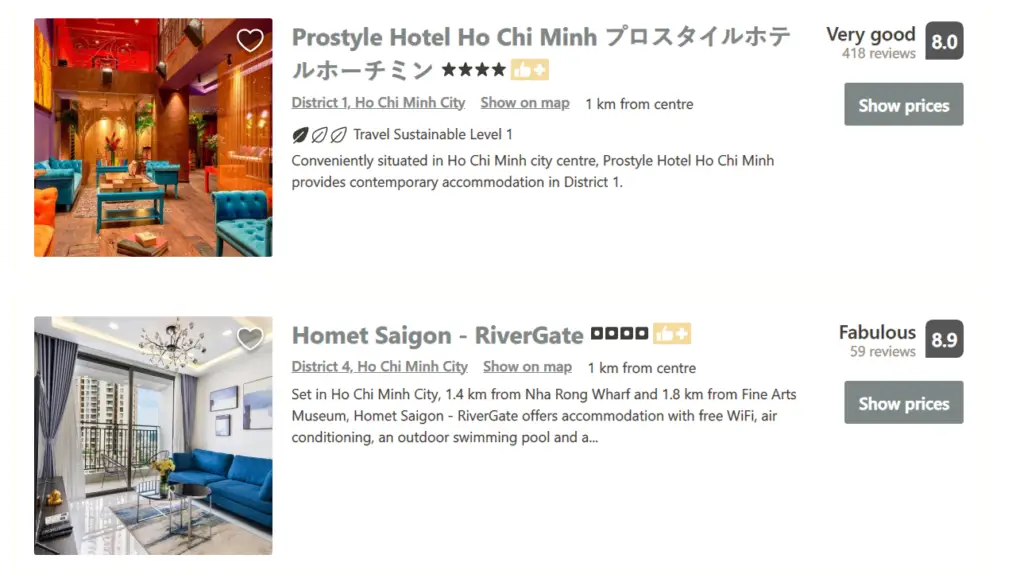**Detailed Captions for Hotel Listings on a Travel Website**

*First Listing: Pro Style Hotel Ho Chi Minh*

The image showcases an elegant lobby with modern decor. The lobby features luxurious blue velvet sofas and matching tables, interspersed with vibrant orange sofas, all under high ceilings. Yellow or orange drawstring curtains hang, adding a striking visual element.

To the right of the image, the hotel details are provided:
- **Name:** Pro Style Hotel Ho Chi Minh (also includes Japanese writing)
- **Rating:** Four black stars
- **Icon:** A brown box with a white thumbs up and a plus sign
- **Review Summary:** "Very Good" with a score of 8.0 in a dark gray box
- **Number of Reviews:** 418 reviews
- **Action Button:** A dark gray button labeled "Show Prices" in white font

Additional Information under the hotel name:
- **Location:** District 1, Ho Chi Minh City
- **Distance:** 1 kilometer from the center (with a link to show on map)
- **Sustainability:** Travel Sustainable Level 1, indicated by three leaf-like symbols

Description:
"Conveniently situated in Ho Chi Minh City Center, Pro Style Hotel Ho Chi Minh provides contemporary accommodation in District 1."

*Second Listing: Ho Met Saigon. River Gate*

The image features the interior of a high-rise hotel room. It has a floor-to-ceiling window with views of city high-rises, a blue sofa, a coffee table, and a rug on white floors.

To the right of the image, the hotel details are provided:
- **Name:** Ho Met Saigon. River Gate
- **Rating:** Four black stars
- **Icon:** A yellowish-brown square with a white thumbs up and a plus sign
- **Review Summary:** "Fabulous" with a score of 8.9 in a gray box
- **Number of Reviews:** 59 reviews
- **Action Button:** A gray button labeled "Show Prices" in white font

Additional Information under the hotel name:
- **Location:** District 4, Ho Chi Minh City
- **Distance:** 1 kilometer from the center (with a link to show on map)

Description:
"Set in Ho Chi Minh City, 1.4 kilometers from Nga Rung Wharf and 1.8 kilometers from Fine Arts Museum, Ho Met Saigon. River Gate offers accommodation with free Wi-Fi, air conditioning, an outdoor swimming pool, and more."

This detailed caption now presents the information in a clear and structured manner, capturing all the key elements of each hotel listing.